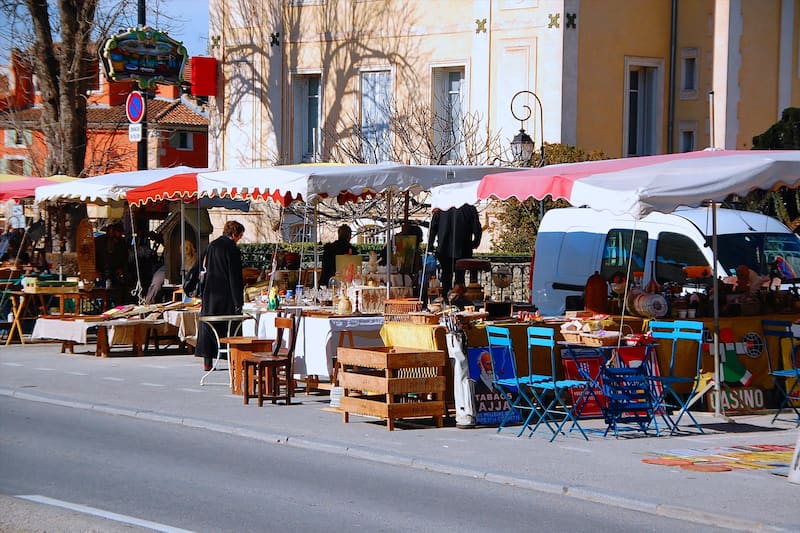The image captures a bustling street market scene with vendor booths set up along the far sidewalk, viewed from across the street on a pavement foreground. The five booths, seemingly operated by antique and collectible dealers, are arranged side by side, stretching into the distance under a series of awnings. Various tables are loaded with an assortment of antiques, glassware, and miscellaneous items, with several chairs placed around them. Behind the booths, a blue and white van is parked, adding to the eclectic ambiance. Vendors are seen minding their tables, engaging in conversations and sales, while a solitary customer, clad in a dark coat, stands central with her back to the camera, inspecting the wares. In the background, there are buildings that frame the lively scene, providing a glimpse into the everyday hustle and bustle of this charming street market.